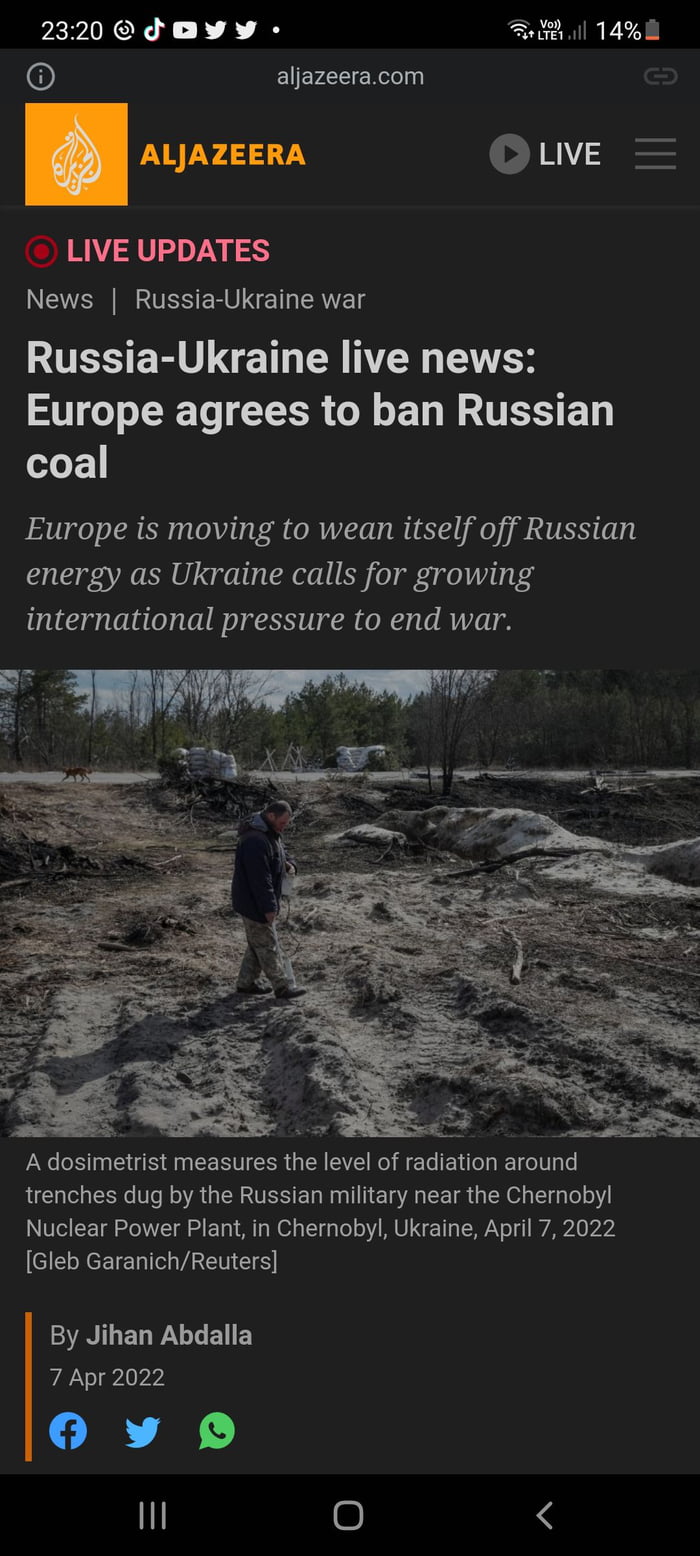Displayed is a mobile version of the Al Jazeera website. The top of the screen shows the URL, aljazeera.com, indicating that this is the browser version and not the Al Jazeera app. The section featured is dedicated to live updates on the Russia-Ukraine war. The main headline reads, "Russia-Ukraine War Live News: Europe Agrees to Ban Russian Coal." The byline elaborates, stating that "Europe is moving to wean itself off of Russian energy as Ukraine calls for growing international pressure to end the war." Below the headline, there is an image likely depicting a scene from Ukraine, complete with a descriptive caption detailing the context of the war situation.